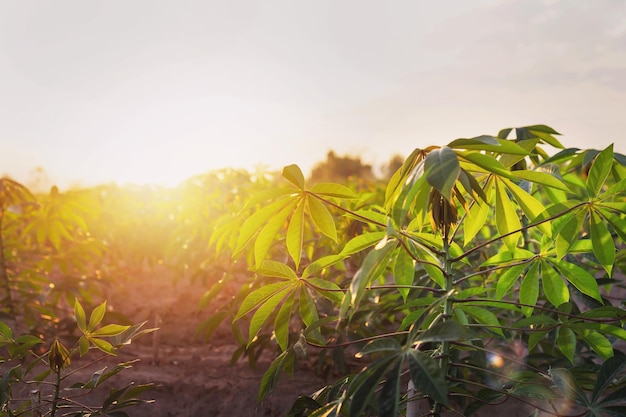The photo captures an outdoor scene in a field during the early morning as the sun begins to rise, casting a bright, diffused light that makes the sky appear grayish-white with hints of purple in the top right corner. The field is populated by a green leafy plant that dominates both the foreground and stretches into the distance. Each plant is approximately a foot to a foot and a half tall, featuring stems with clusters of five smooth-edged leaves. The bottom left of the image shows patches of brown dirt, while the bottom right is filled with green leaves extending from thin stems. Overall, the sky's brightness creates a serene ambiance, suggesting a clear and tranquil morning with minimal clouds.